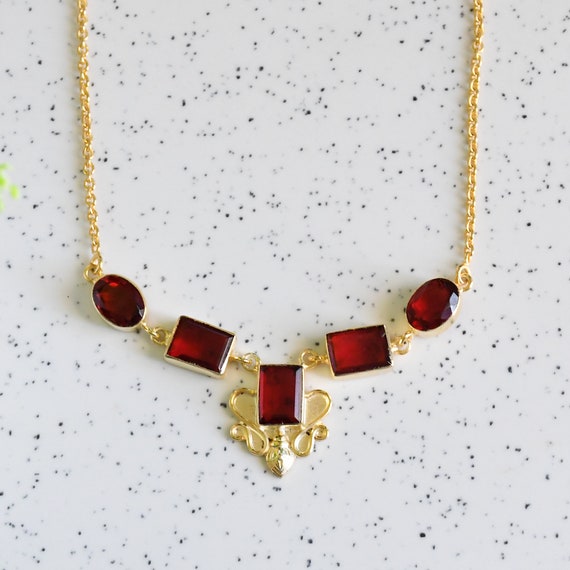This square photograph captures a close-up view of a beautifully crafted gold necklace adorned with deep red gemstones, likely rubies or garnets. The necklace, resting on a white surface speckled with black or gray dots, features a total of five gemstones linked in a symmetrical design. Starting from the outer edges, there are two oval-shaped stones, followed by two horizontally rectangular stones. The centerpiece is a vertically oriented rectangular gemstone, which is taller than it is wide and framed with an ornate gold setting. The strands of the necklace extend from the upper left and upper right corners of the image, converging below in the middle, creating an elegant and balanced composition.